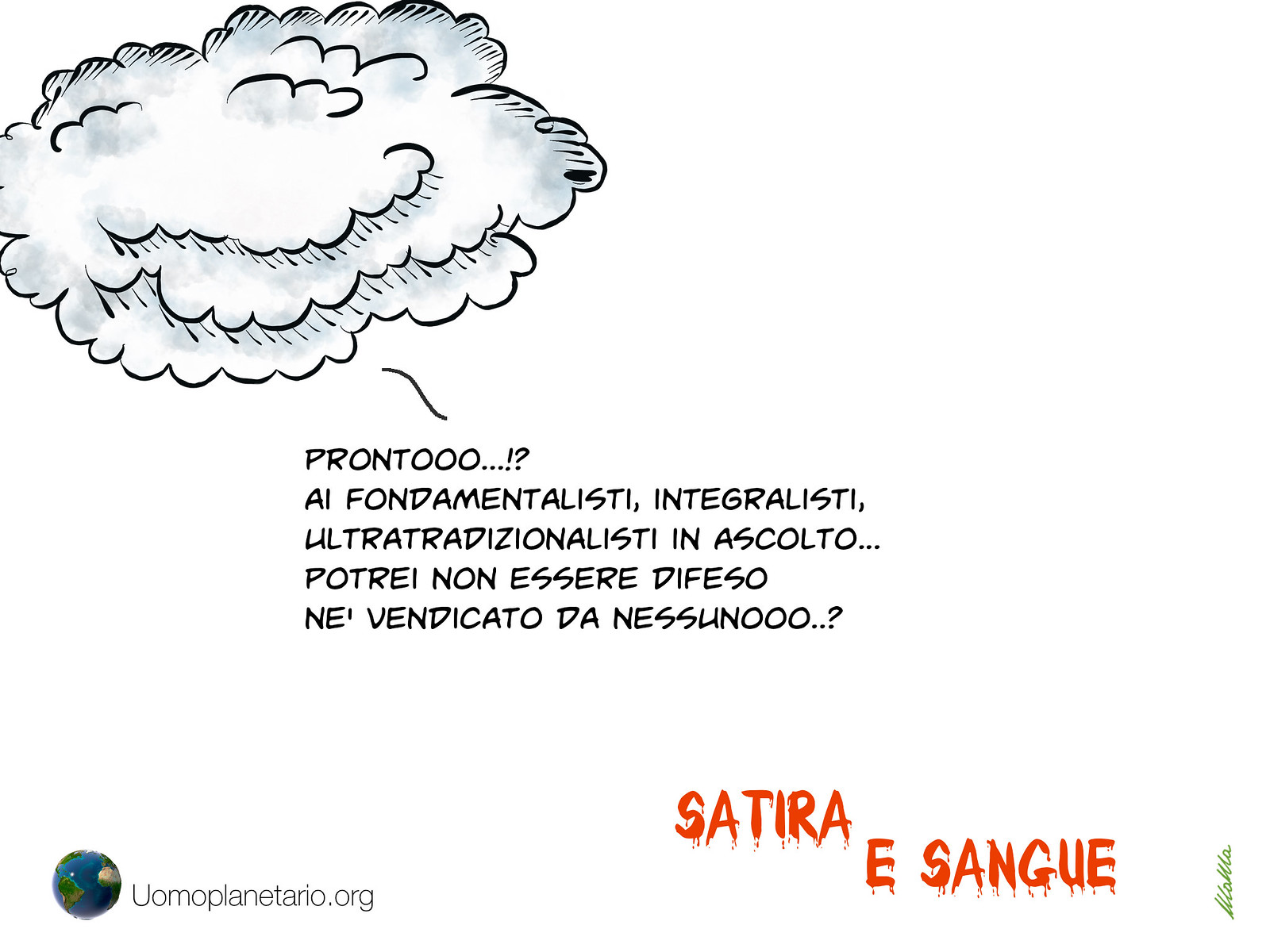The image is a cartoon drawing with a completely white background. In the top left-hand corner, there is a large, fluffy cloud outlined in black and filled with white and light gray accents. Emerging from the cloud is black text in Italian that reads, "Pronto, a fondamentalisti, integralisti, ultra-tradizionalisti, in ascolto, potrei non essere difeso, ne vendicato, de nessuno." In the bottom left corner, there is a colored illustration of a globe with the text "uomoplanetario.org" next to it. In the bottom right corner, there are orange-red letters that spell out "satira e sangue". Additionally, there appears to be an unreadable signature in the bottom right corner.